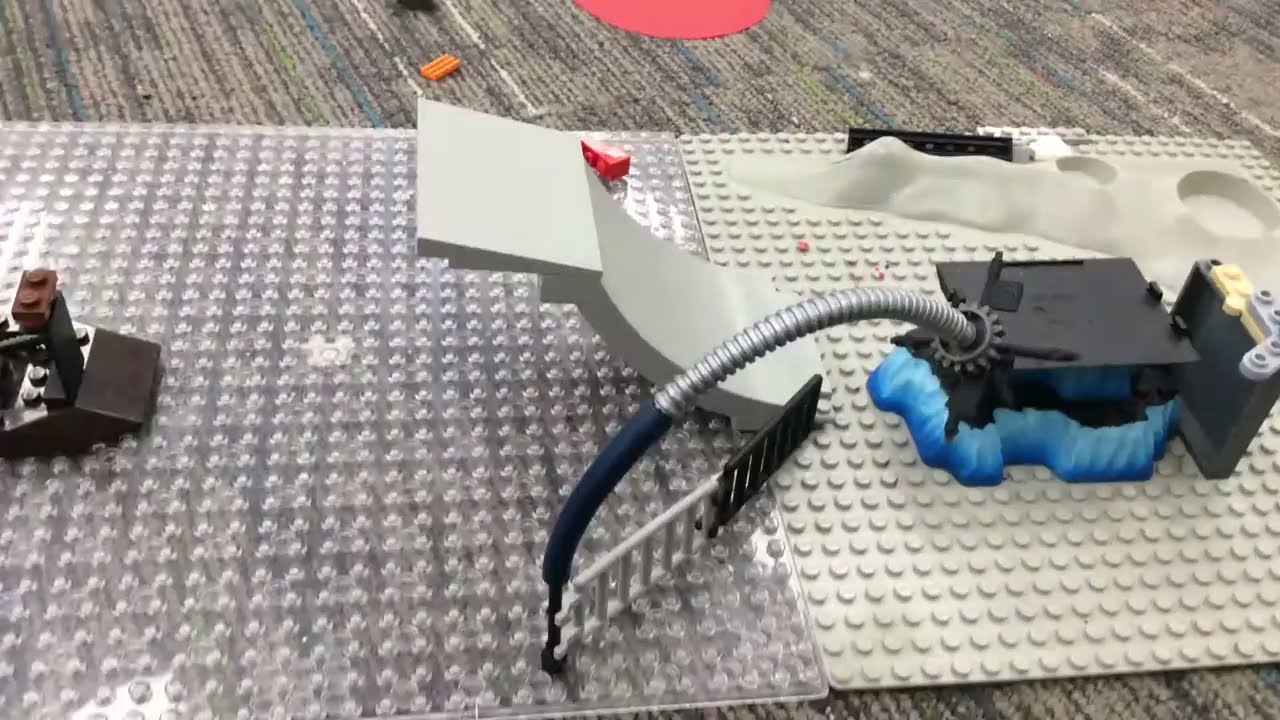The image is a detailed color photograph of Lego pieces arranged on a beige striped carpet with thin stripes of darker gray, green, and blue. The photo is horizontally aligned and shows two large Lego base plates side by side but not connected. On the right, there is a really large square gray Lego plate, while on the left, there's a clear one. Scattered around are various smaller Lego builds and pieces of paper.

On top of these plates are two Lego ladders, one gray and one black, which are connected. Attached to the end of the gray ladder is a blue tube connected to a spiral narrow gray piece and another tube. This assembly is situated on the large gray Lego plate and appears to be part of a Technic set that has a flat black top and a blue bottom.

In the middle, roughly between the two base plates, there is a white Lego ramp. Behind the main assembled object, which includes the hose and tube, is a plastic configuration resembling mountains with cutout holes, along with a black vertical plastic piece that has a yellow and gray top. On the left side of the image, there's a black unit that looks like a controller.

Lastly, there is a red circular object at the top, enhancing the complexity and detail of the scene. The overall style of the image is photographic representational realism, capturing the intricate early stages of what might be an ice-themed Lego construction set.